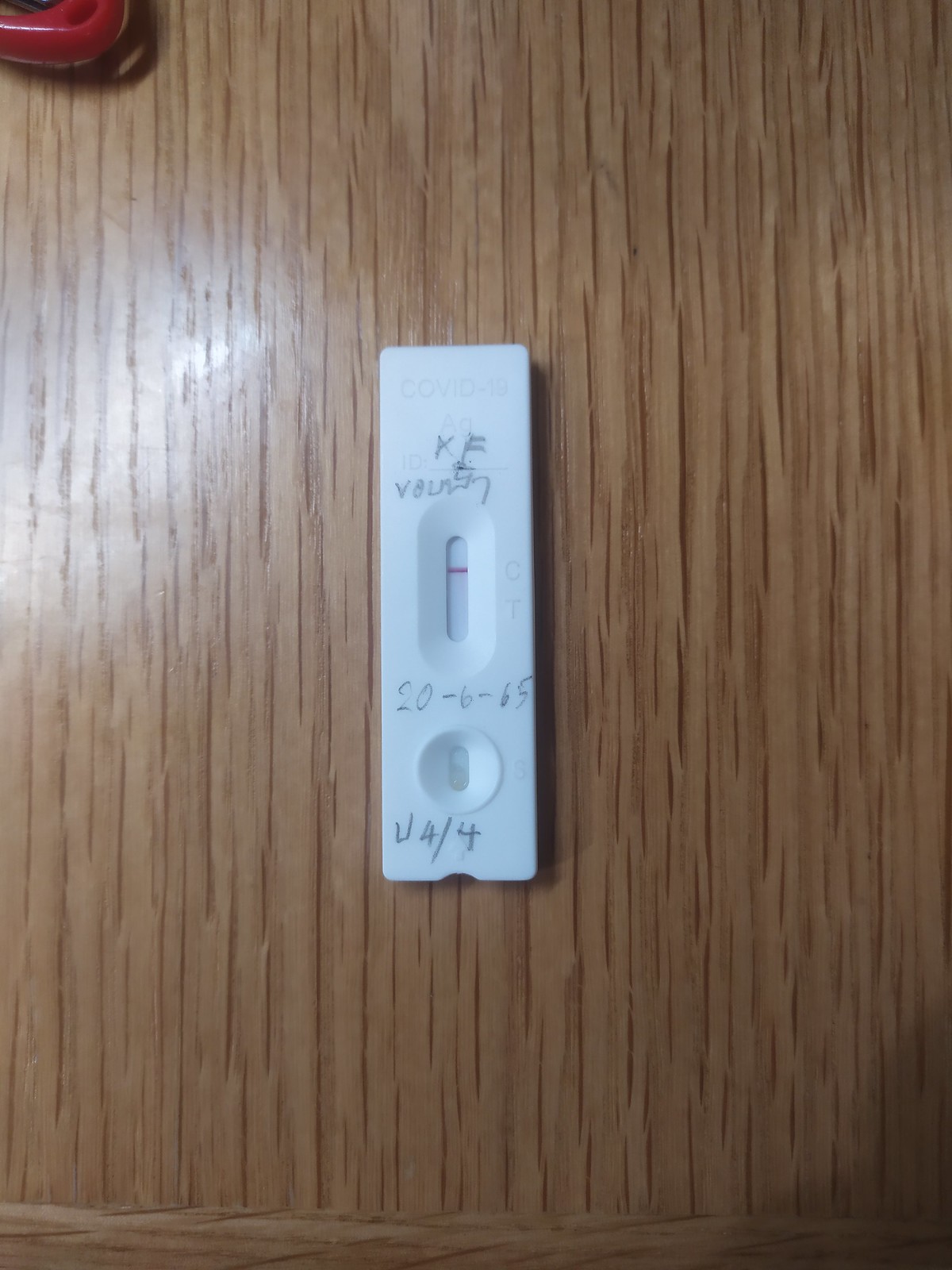Indoor color photograph taken from above, showcasing a hardwood surface, possibly a countertop or table, with a light tan wood grain running vertically. Centrally positioned on the surface is a rectangular plastic medical testing device, likely used for blood testing. The device features a vertical, rectangular thin window with a red horizontal line positioned in the upper half. To the right of this window, faint letters are visible: a "C" at the top and a "T" below it, both in uppercase.

Above this window, written in pen or pencil, are the capital letters "KF," followed by a partially legible phrase "VOLA something Y." Below this text is a date inscribed as "20-6-65." In the lower section of the device, there is a circular opening accompanied by a smaller vertical oval slot, both white. Beneath this, also written in pen or pencil, are the characters "U4/4." Just beside the circle, the letter "S" is faintly visible. The light source, coming from the left, casts a subtle shadow to the right of the device, enhancing the three-dimensional quality of the image. This setup suggests the device is intended for a blood sample or blood test.